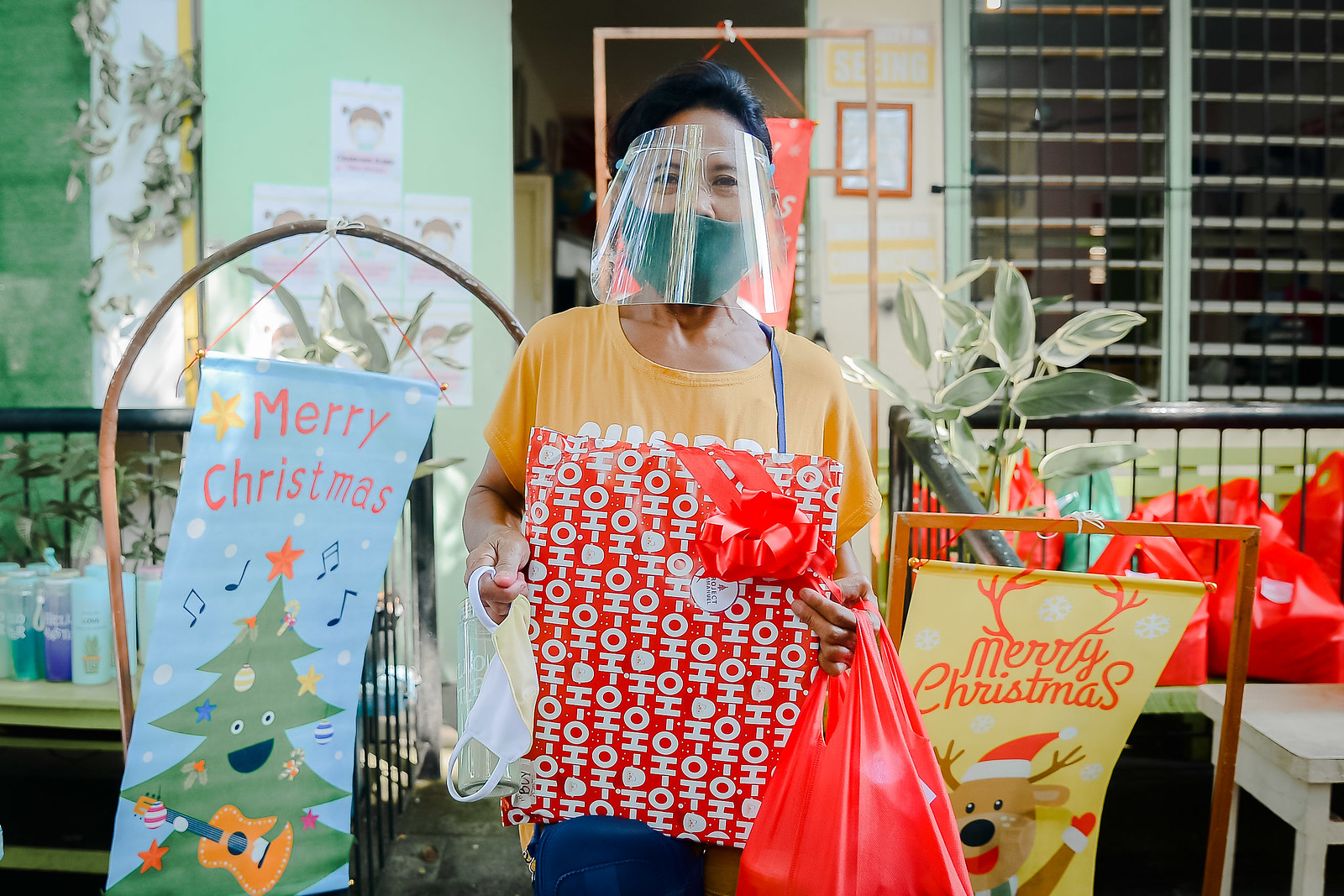A color photograph in landscape orientation captures a person, likely a woman, standing centrally in a room adorned with vibrant Christmas decorations. She wears a yellow short-sleeve blouse and an orange apron, with a blue face mask covered by a clear plastic shield. Holding a red package emblazoned with "HO HO HO" in white letters, she epitomizes the festive spirit amidst the height of COVID-19 precautions. The backdrop features contrasting banners: a blue "Merry Christmas" banner on the left and a yellow one on the right. Additional holiday cheer is provided by a Christmas tree, reindeer decoration with a hat, and smiling red gloves. Behind her, a green wall and red bags are visible, suggesting the bustling environment of a store. The photograph appears to be an interior shot with photographic realism, capturing the essence of a holiday shopping experience during a pandemic.